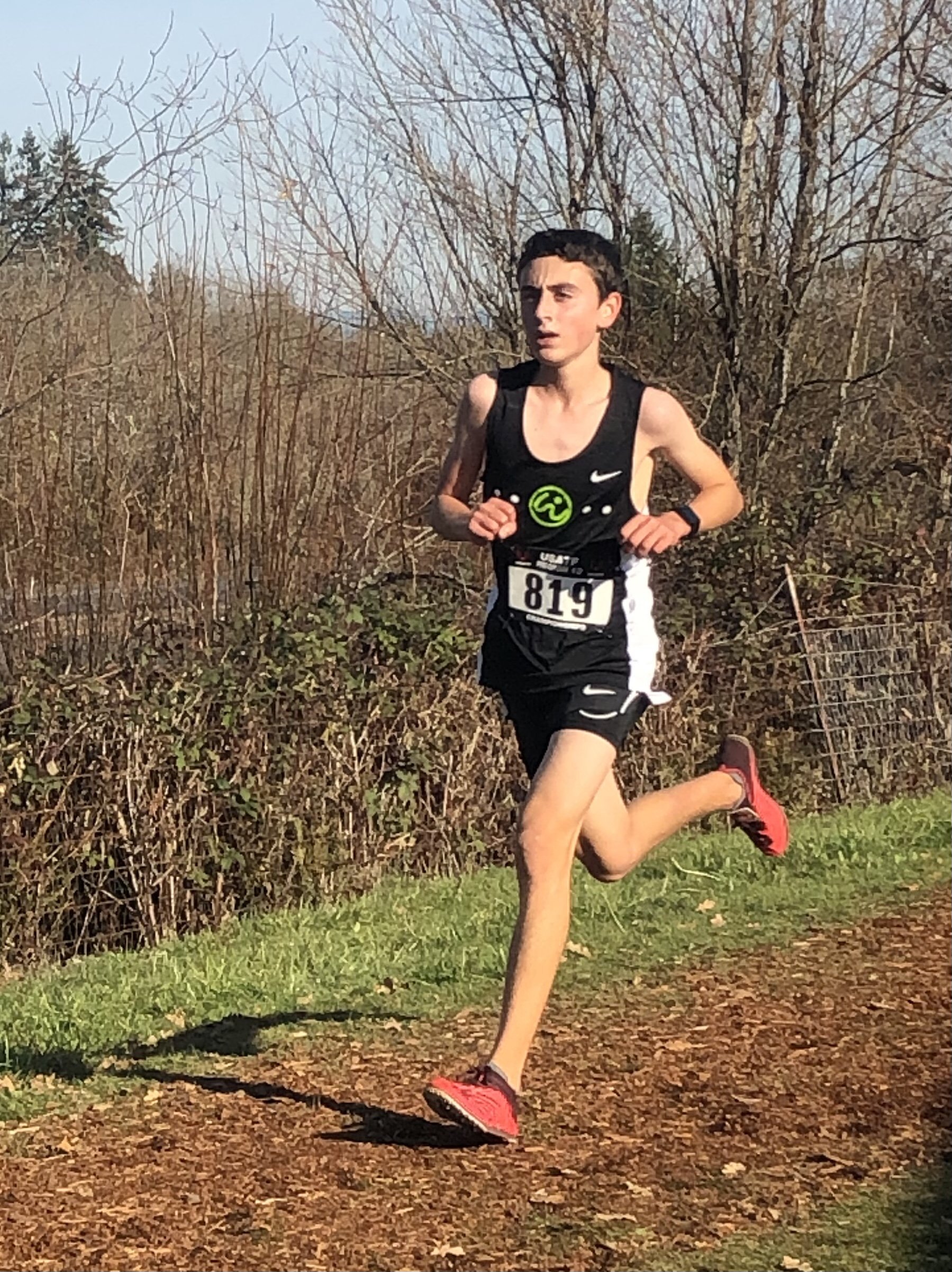In this vivid image, a Caucasian teenage boy, appearing about 15 years old, is captured running in a cross-country race on a dirt trail. He sports a focused, serious expression as he advances along the trail, clad in dedicated running gear. The boy is dressed in a black sleeveless shirt with a white Nike swoosh logo on the chest and a number 819 displayed prominently in a rectangular white section on his stomach. Complementing his top, he wears black running shorts, also adorned with a Nike swoosh, and bright red running shoes. A black watch is fastened to his wrist. His short black hair contrasts with his rather pale complexion. The trail, a browned-out section of ground about four feet wide, cuts through a field. To his right, a field dense with leafless vegetation stretches out, painting a stark yet serene backdrop to his strenuous effort.